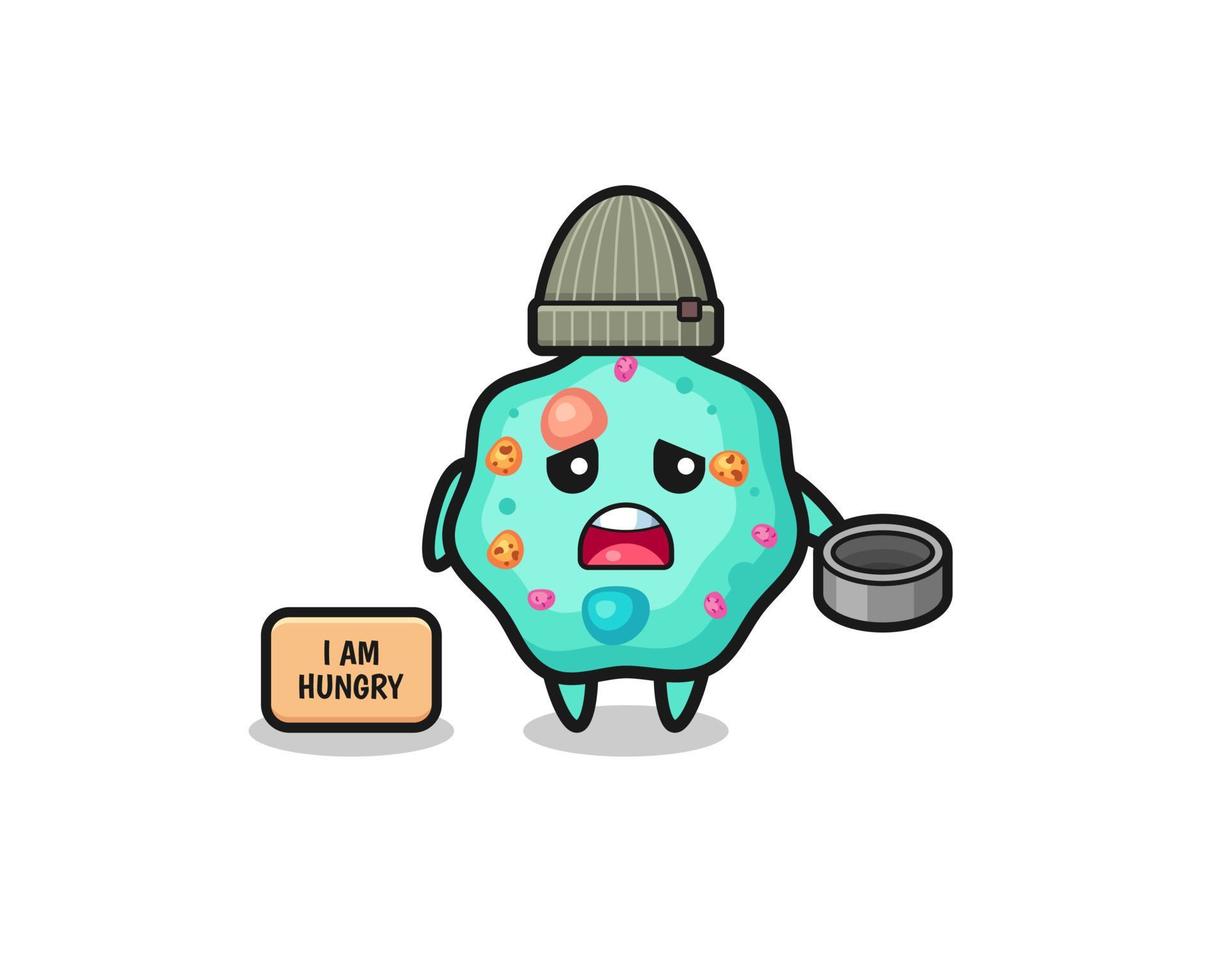The image is a cartoon-like graphic design featuring a light blue, anthropomorphized amoeba-like blob with a sad, grumpy face, complete with visible teeth and tongue. The blob has two arms and two legs and is adorned with several spots, including ones resembling chocolate chip cookies and a couple in blue and pink. Perched on its head is a gray knit ski cap with white vertical stripes and a small brown emblem. In one hand, the blob holds an empty gray food bowl, and on the ground nearby, a round-shadow-casting orange sign reads, "I am hungry." The scene is set against a white background, with the entire illustration rendered in a simple, thick-lined, clip art style that lends a chunky and somewhat shadowed appearance to the design.